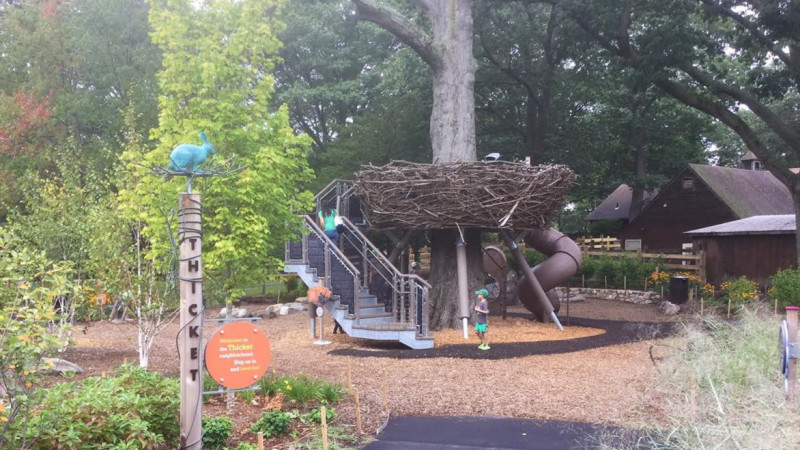In this detailed image, a playground with a natural theme is situated within a nature preserve or park area known as "The Thicket." The focal point of the playground is a massive tree with a large nest-like structure made from intertwined branches perched about 10 feet off the ground, encircling the trunk. Access to the nest is provided by stairs, while a spiral slide offers a fun descent. 

A signpost to the left prominently displays the word "Thicket" in brown letters, adorned with wrapped wood branches and topped by a platform featuring a blue rabbit. Despite an orange sign with yellow and white writing on the post, the text isn’t clear. Surrounding the nest area are both paved pathways and patches of asphalt.

In the scene, a lady in a green top and blue pants with a black and white purse is climbing the steps towards the nest, accompanied by a young boy at ground level. The backdrop features tall, leafy trees along with some smaller green trees. On the right side, there is an old, country-style brown house with a wooden fence and garden plants, contributing to the picturesque, family-friendly environment of the playground.